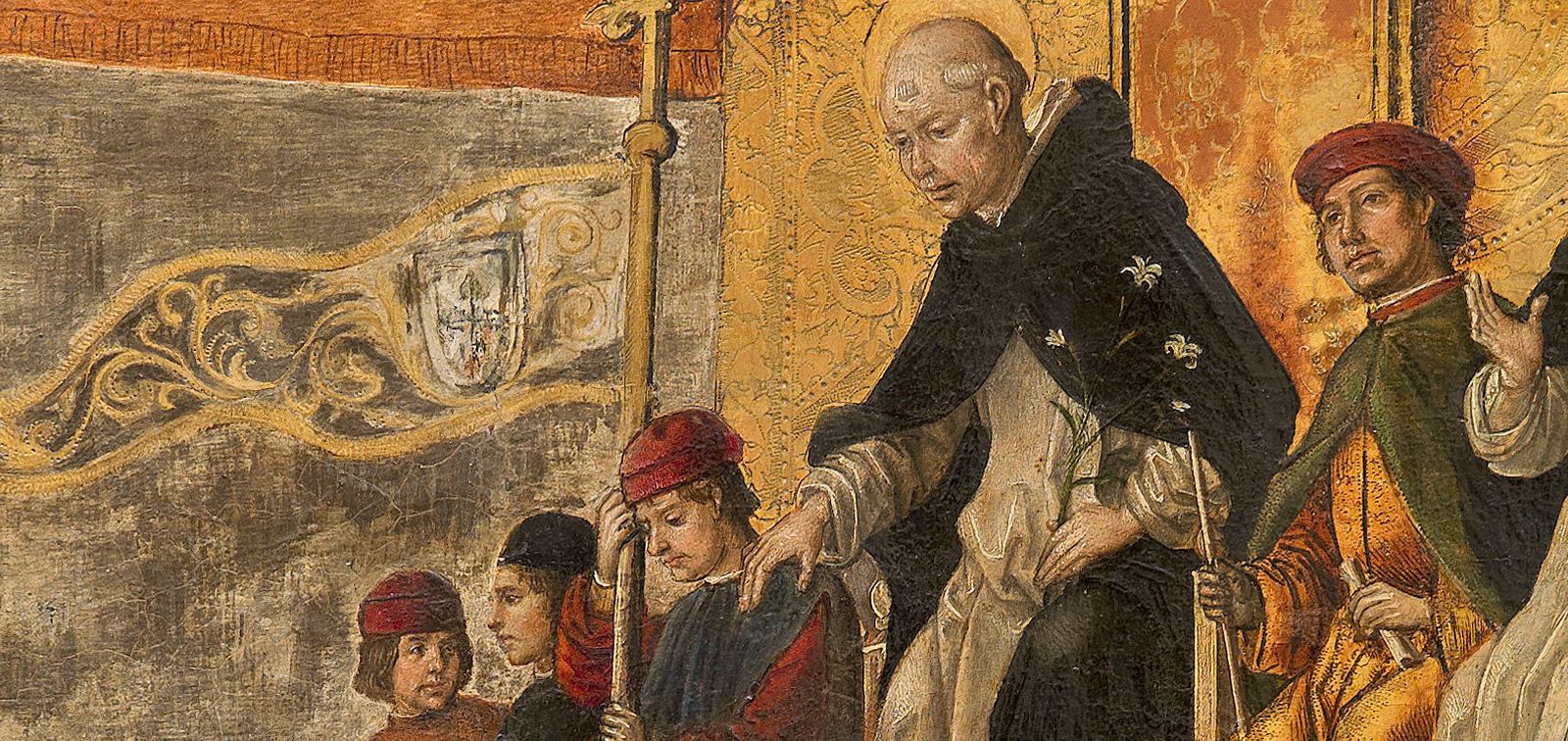This detailed painting appears to depict a scene from the Spanish Inquisition. At the center of the artwork stands an older man, bald-headed, exuding authority. He wears a black cloak over a cream-colored robe and holds a green stem with small white flowers. Beside him, likely his servant, is a man in a gray robe with a striking red hat and shirt who is holding a large golden flag adorned with a country crest. To the older man's left is another figure clad in a green cloak and red hat, holding a piece of paper and a rod, suggesting he might be a messenger. On the far right, two additional men in red hats seem to exchange concerned glances. The background is rich with earthy tones, including a mix of brown, yellow, and bronze hues. A golden wall with ornate designs is prominent, contrasting with a gray section on the left of the painting. The fine line work in the illustration intricately conveys texture and age, adding depth and detail to the characters and the setting.